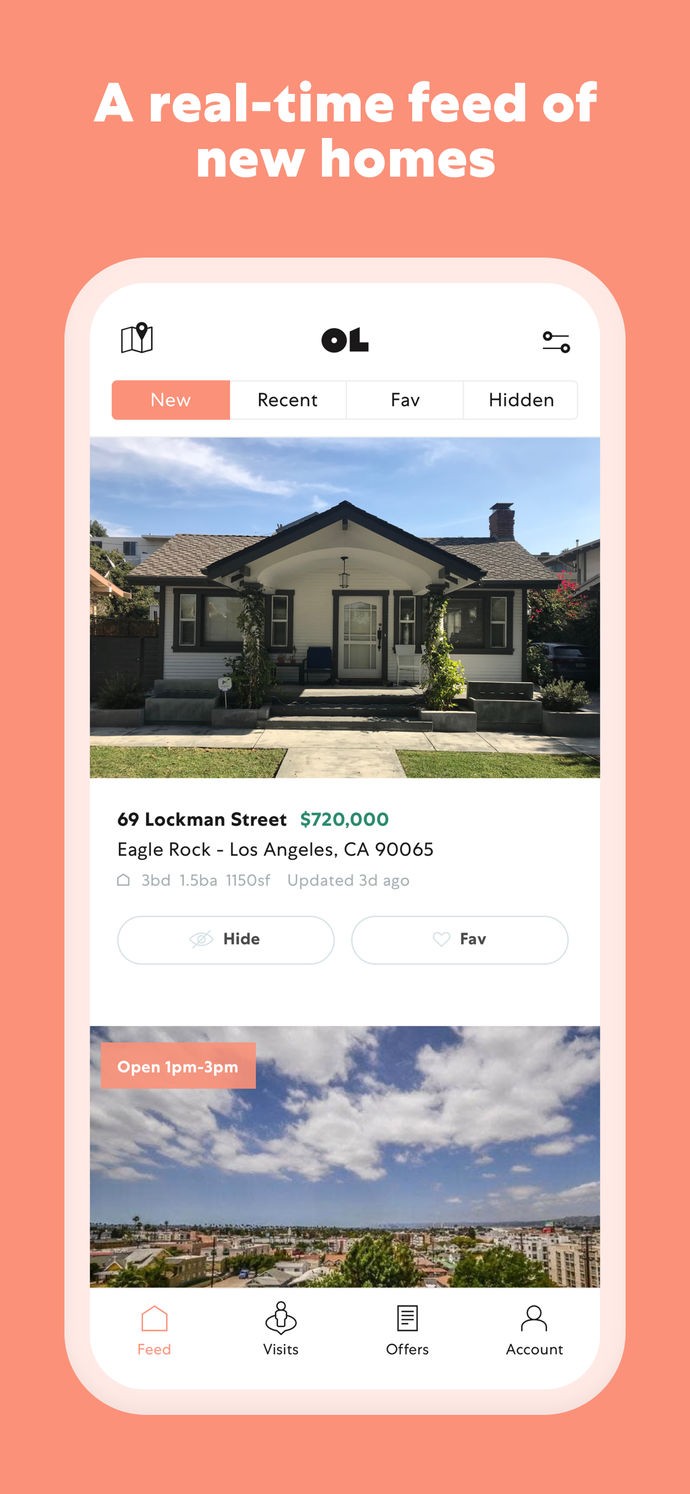The image displays a white-colored cell phone set against a background with a gradient transitioning from orange to pink hues. The phone's screen showcases various elements in a well-organized layout. At the top, bold white text reads "A real-time feed of new homes."

The perimeter of the phone is outlined in a subtle pink shade, while the interior screen area is primarily white. In the upper left corner, there is a small map icon. Centrally located at the top of the screen, bold black letters "OL" are displayed, and in the upper right corner, a filter icon is visible.

Below these elements, a navigation menu features the options "News," "Recent," "Fave," and "Hidden," with "New" prominently highlighted in an orange color. Beneath this menu, an image of a white and brown colored house is featured. Text accompanying the image detail the property: "69 Lachman Street, $720,000. Eagle Rock, Los Angeles, California, 90065," followed by specifications including "three-bedroom, 1150 square feet." An additional note mentions that the listing was updated three days ago, and options to "hide" or "favorite" the listing are presented.

Further down, an image of a blue sky with scattered clouds indicates an open house time of "1PM to 3PM." At the bottom of the screen, navigation options including "Feed," "Visits," "Offers," and "Account" are available.